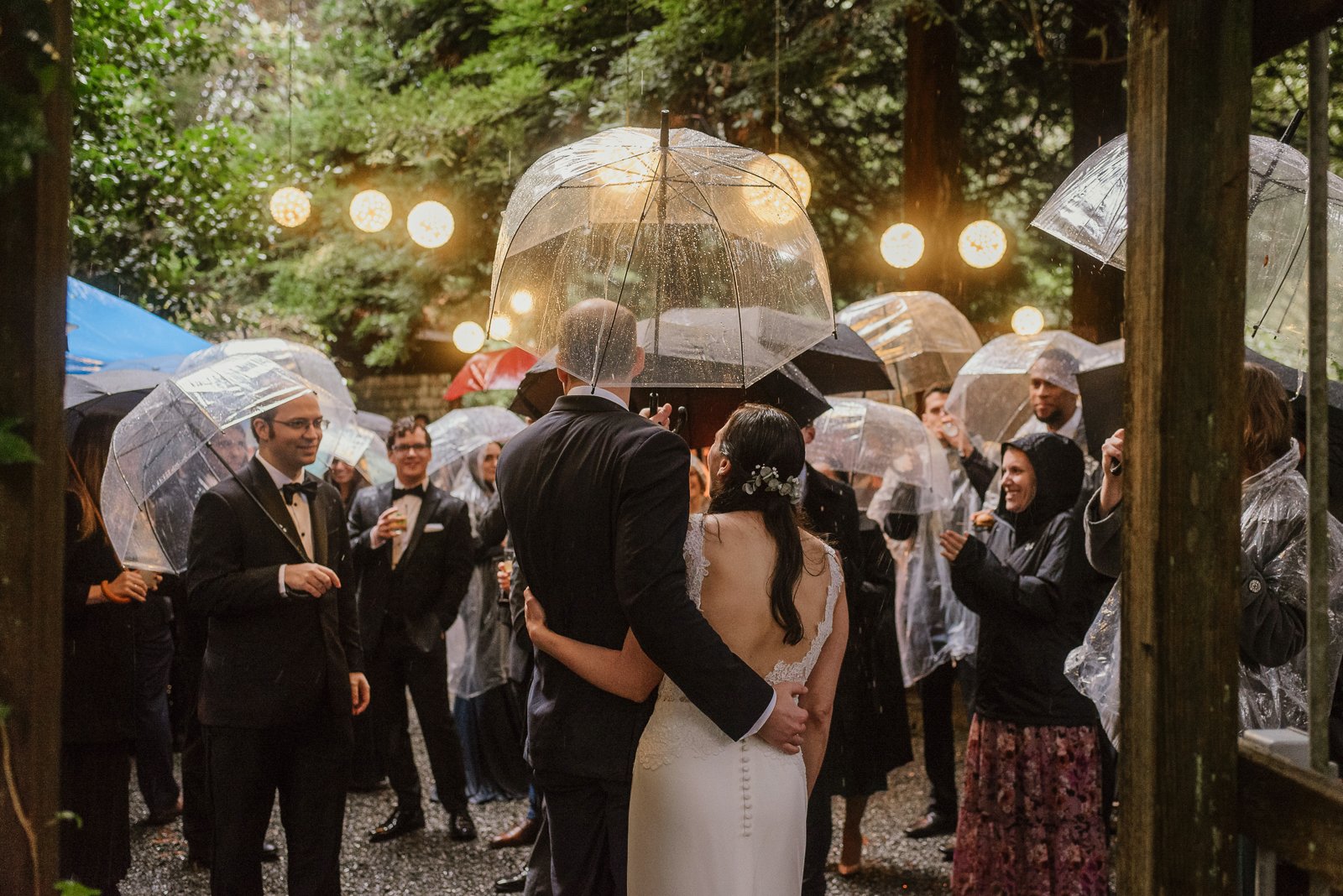In this vibrant outdoor wedding photograph, the bride adorned in a white dress, with a garland or ribbon in her hair, stands closely with the groom, who is dressed in a black suit. They are positioned at the center with their backs to the camera, each with an arm wrapped around the other, facing an assembled crowd. The gathering, set in a lush garden with a gravel surface and surrounded by green trees, has a festive yet serene atmosphere accentuated by hanging white orb lights indicating early evening. Despite the rain, the celebration continues with most guests holding translucent plastic umbrellas provided by the venue. Among the attendees, men in tuxedos are prominently visible, alongside women in raincoats and long dresses, such as a woman in a black coat with a hood and pink dress. The crowd's happy demeanor suggests a joyous wedding celebration amidst nature’s embrace.